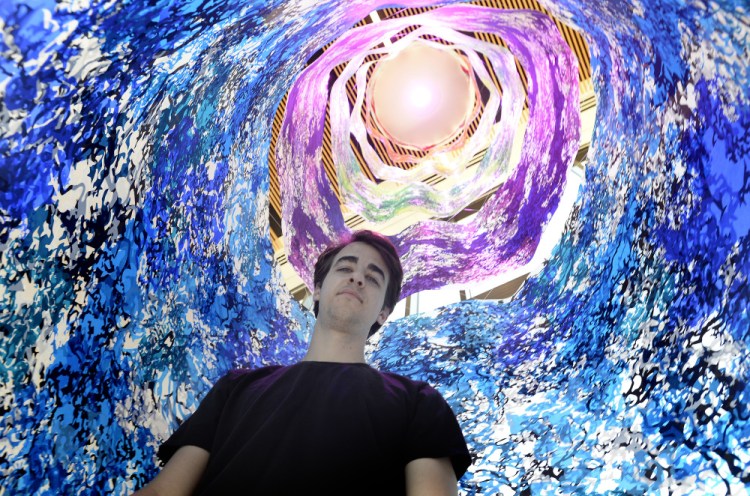In this captivating photograph, we see a man, appearing happy with a smirk, seemingly taking a selfie from a low angle. The perspective is from the ground looking up, capturing the intricate layers of a vibrant art installation that surrounds him. At the center of the image is the man, identifiable by his ear-length dark brown shaggy hair and a black t-shirt with short sleeves. 

He is enclosed within a cylindrical arrangement of colorful crystal walls, starting with a striking blue layer at the bottom that frames the edge of the picture. Above him, the art transitions into a ring of purple, followed by layers with diverse shades of green and white, dotted with hints of light blue and teal. These layers extend upward toward the ceiling, which features yellow vertical lines converging at the top around a large white dome light, resembling a giant pearl or lamp cover. The overall effect is a mesmerizing display of color and light, with the man at its vibrant core, smiling against this dynamic, multi-layered backdrop.